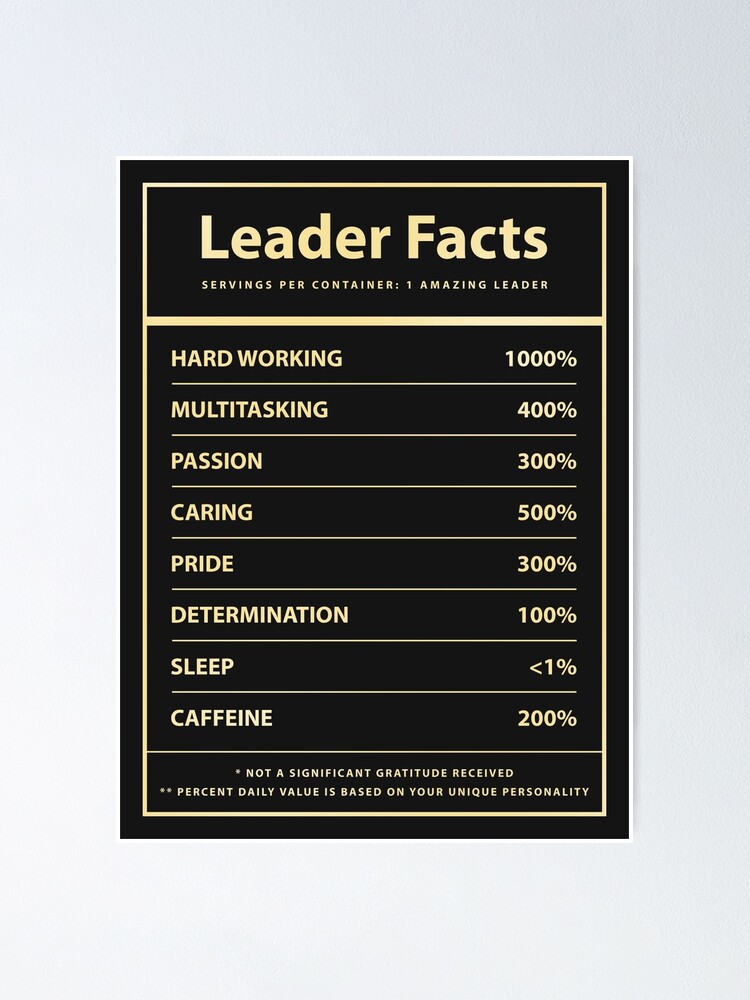The image is a vertical graphic design roughly 5 inches wide by 8 inches tall, set against a gray background with a thin white border. Inside this, a black rectangular layout features a yellow (gold) border. At the top, in gold font, the text reads "Leader Facts" with the subtitle "Servings Per Container: One Amazing Leader" beneath it. A yellow horizontal line separates this header from a detailed list of leader characteristics displayed within the black box: "Hard-working 1,000%, Multitasking 400%, Passion 300%, Caring 500%, Pride 300%, Determination 100%, Sleep < 1%, Caffeine 200%." At the bottom, an asterisk notes, "Not a significant gratitude received," and two asterisks indicate, "Percent daily value is based on your unique personality." The design does not contain any attribution to a website or external source.